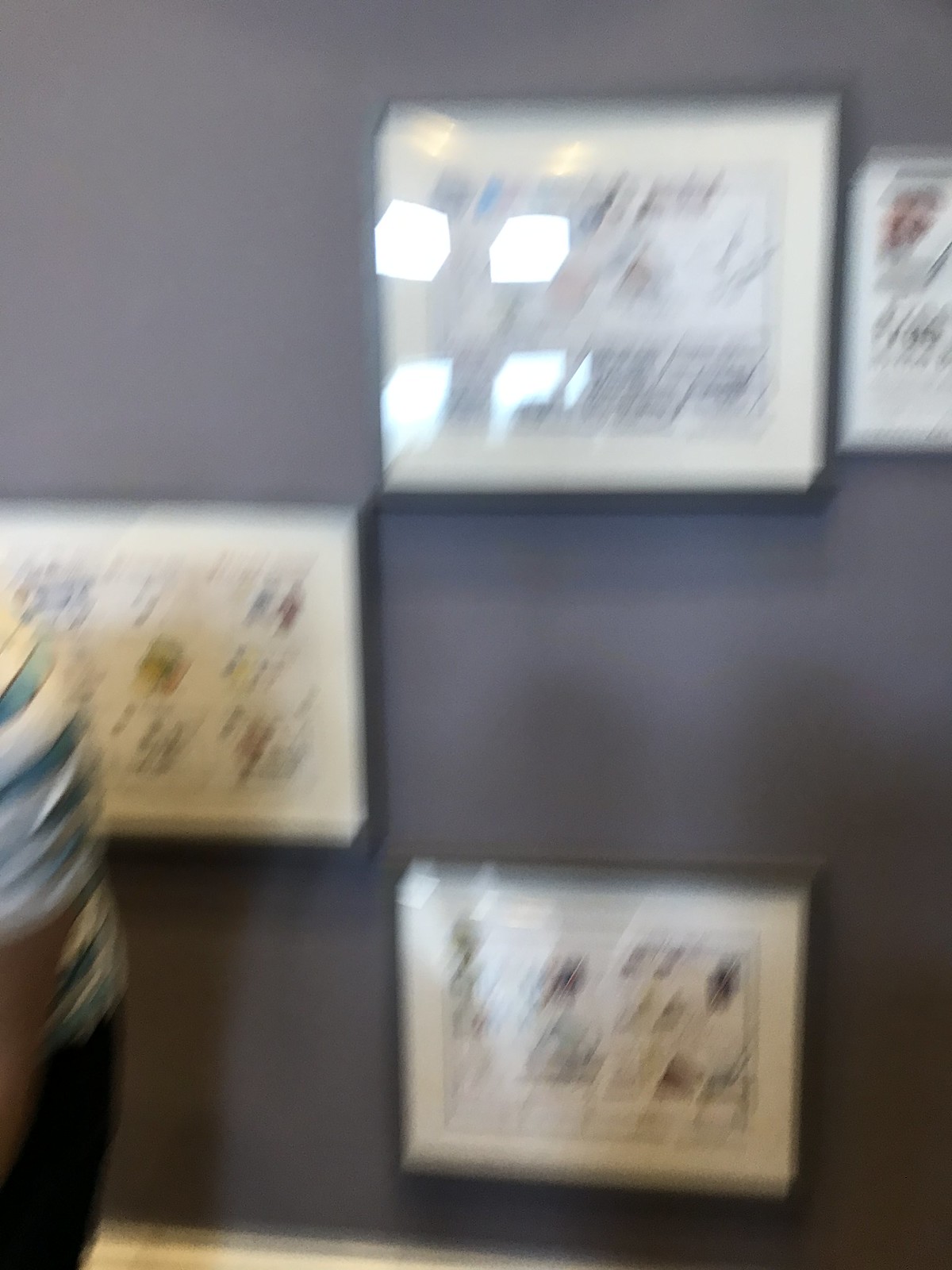The photo depicts a dark gray wall adorned with four framed portraits, all featuring dark frames and white mattes. Due to significant motion blur, the images within the frames are indiscernible, though there's a suggestion that they might be flower portraits. The artwork is arranged with one piece at the top right corner and another directly below it, while the third is to the left, situated between the other two. Near the bottom of the wall is the fourth frame. Additionally, there is part of a person on the left side of the image, wearing a white and turquoise striped short-sleeve t-shirt and dark pants, seemingly bending over. The photo has a noticeable glare, likely from artificial light, contributing to the overall blurriness of the scene.